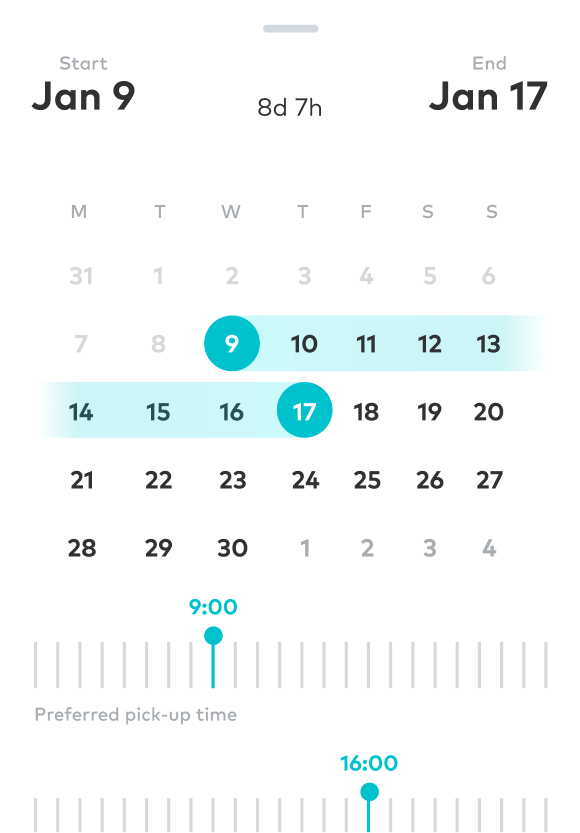The image displays a detailed calendar interface. The main focus is on a timeframe starting from January 9th, noted in black text, and ending on January 17th, also in black text. The 9th is distinctly highlighted in blue, while both the 9th and 17th are accentuated with greenish highlights and blue circles around the dates. 

The calendar visual begins on Monday, the 31st, and extends through the rest of the month, also transitioning into the subsequent month, though only the key dates remain highlighted. 

Below the calendar, there are two line graphs marked with specific times: one at 9:00 AM and the other at 4:00 PM (1600), both rendered in blue with grey dashes indicating potential variability. These times are labeled as preferred pick-up times, suggesting an ideal window for actions though not restricting flexibility outside these times. 

Overall, the calendar and graph combination visually communicate a defined start and end period, with emphasized dates and suggested optimal times for engagement or pickups.